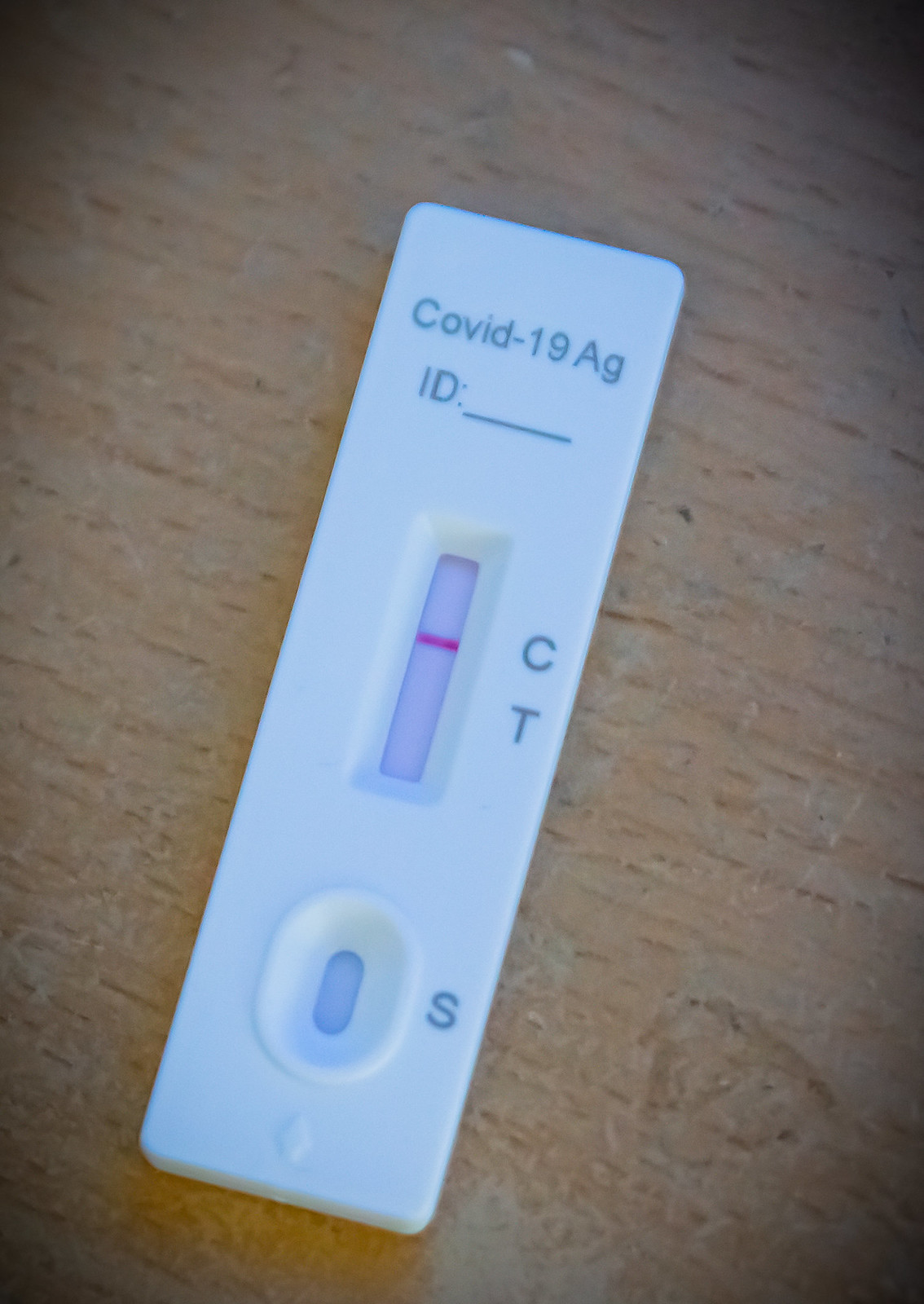This photograph showcases a COVID-19 antigen test taken in portrait mode. The test kit, a long and narrow white plastic device, is placed at an angle on a light-colored wooden surface, possibly a countertop or table. The wooden surface has a distinct water stain visible in the bottom right corner. 

The test kit is labeled "COVID-19 AG" in light blue text at the top. Below this, there is an indented rectangular viewing window, which displays a single red line next to the letter "C," indicating a control line. The letters "C" and "T" are marked to the right of the viewing window, where "C" stands for control and "T" stands for test. The presence of the line next to "C" suggests that the control indication is correct, but the test result cannot be inferred from this line alone.

Near the bottom of the test, there is an oval-shaped indentation labeled "S," likely the sample application area. At the very bottom of the kit, there is a small bump in the plastic, which may serve as a tactile feature or grip area.

This detailed composition effectively highlights the essential features and condition of the test, portraying the key elements needed for interpretation, though it stops short of definitively determining the test result from the image alone.